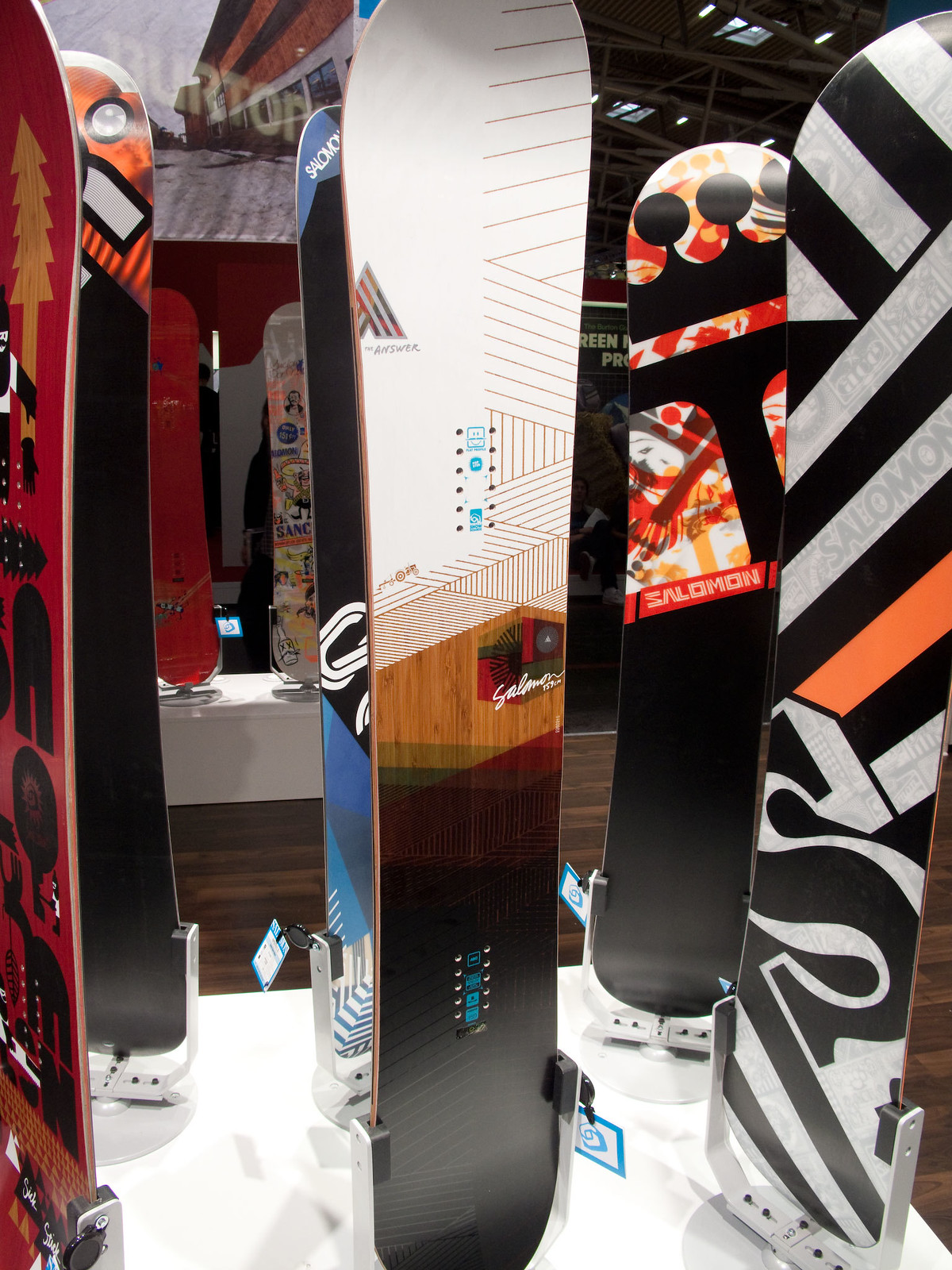This image captures a detailed display of snowboards at a large indoor trade show or conference, with the snowboards standing vertically on a white raised platform about two and a half feet tall. Each snowboard is held in place by metal brackets or U-shaped stands at their ends, allowing their intricate designs to be fully visible at almost eye level. The platform rests on dark brown wood flooring that creates hallways between the rows of snowboards. The designs on the snowboards are highly varied, featuring stripes, multicolors, and technical patterns. Notably, a central snowboard is white with wood accents and a mix of red, green, and black colors, while others include a black and red pattern, a blue, black, and white design, and one with black and white stripes adorned with an orange stripe and the Salomon brand. In the background of this large exhibit hall, more snowboards and different exhibits are visible, including a prominent red structure.